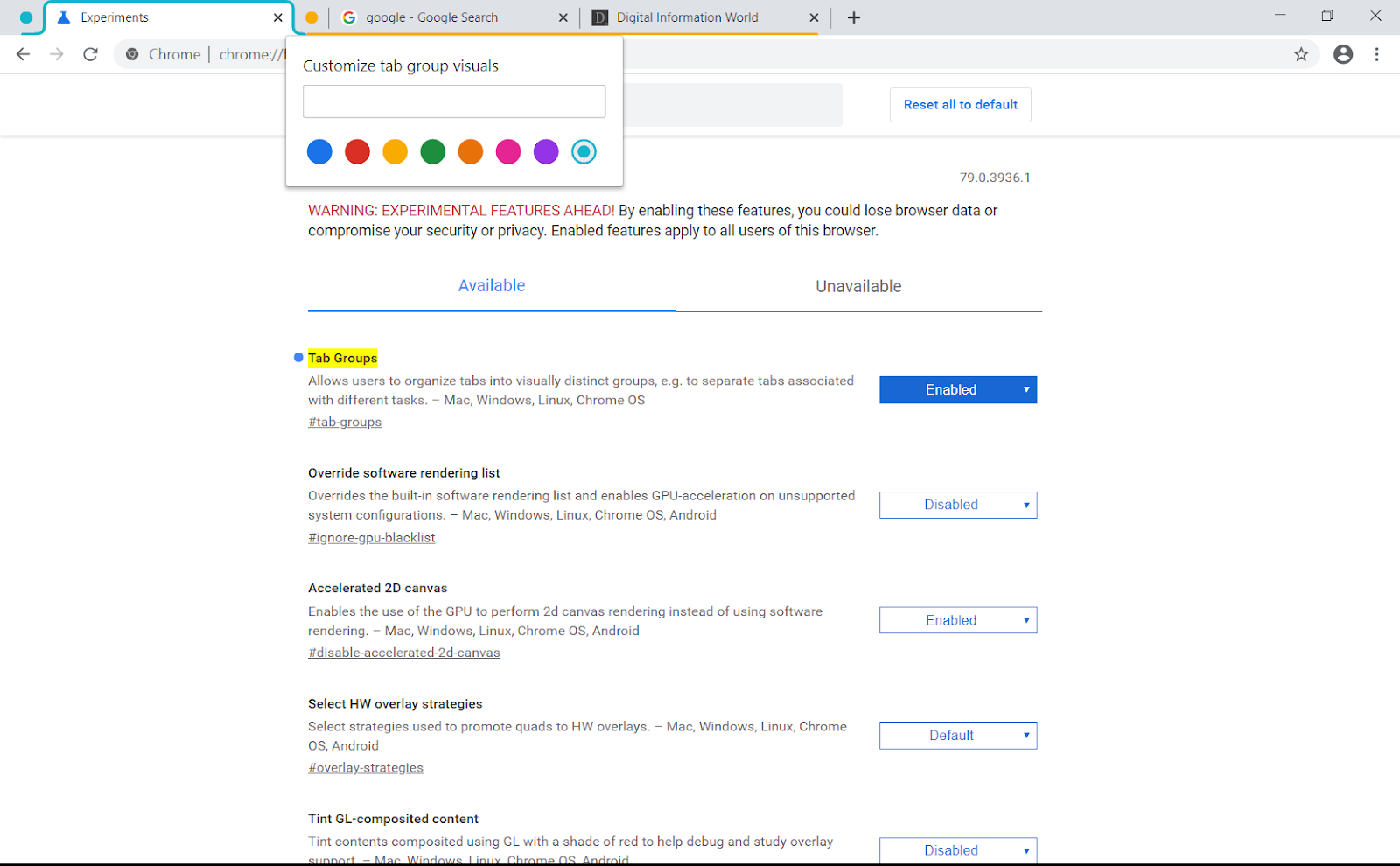In the image displayed on a Chrome browser, the main page is showcasing a feature titled "Customize Tab Group Visual." This feature allows users to organize their tab groups into visually distinct categories using different colors: blue, red, yellow, green, orange, pink, purple, and light green.

A warning highlighted in red states, "Warning: Experimental features are hid." The accompanying description in black text cautions, "By enabling these features, you could lose browser data or compromise your security or privacy. Enabled features may apply to all users of this browser."

Below the warning are two categories, "Available" and "Unavailable," with "Available" being selected and highlighted in blue, while "Unavailable" is greyed out. Within the "Available" category, several experimental features are listed:

1. **Tab Groups:** Allows users to organize tabs into visually distinct groups, each to separate tabs associated with different tasks. This feature is enabled for Mac, Windows, Linux, and Chrome OS, and the "Enabled" button is located on the right side and highlighted in blue.

2. **Override Software Rendering List:** Overrides the built-in software rendering list and enables GPU acceleration on unsupported system configurations. This feature is currently disabled.

3. **Accelerated 3D Canvas:** Enables the use of GPU for 3D canvas rendering instead of using software rendering. This feature is enabled.

4. **Select HW Overlay Strategies:** Allows the selection of strategies used to promote Quartz or HW overlays. This feature is on by default.

5. **Tint GL Composite Content:** Tints GL composite content with a shade of red to help debug and study overlay support. 

The layout and detailed descriptions provide a comprehensive understanding of the customization options and associated risks available through Chrome's experimental features.